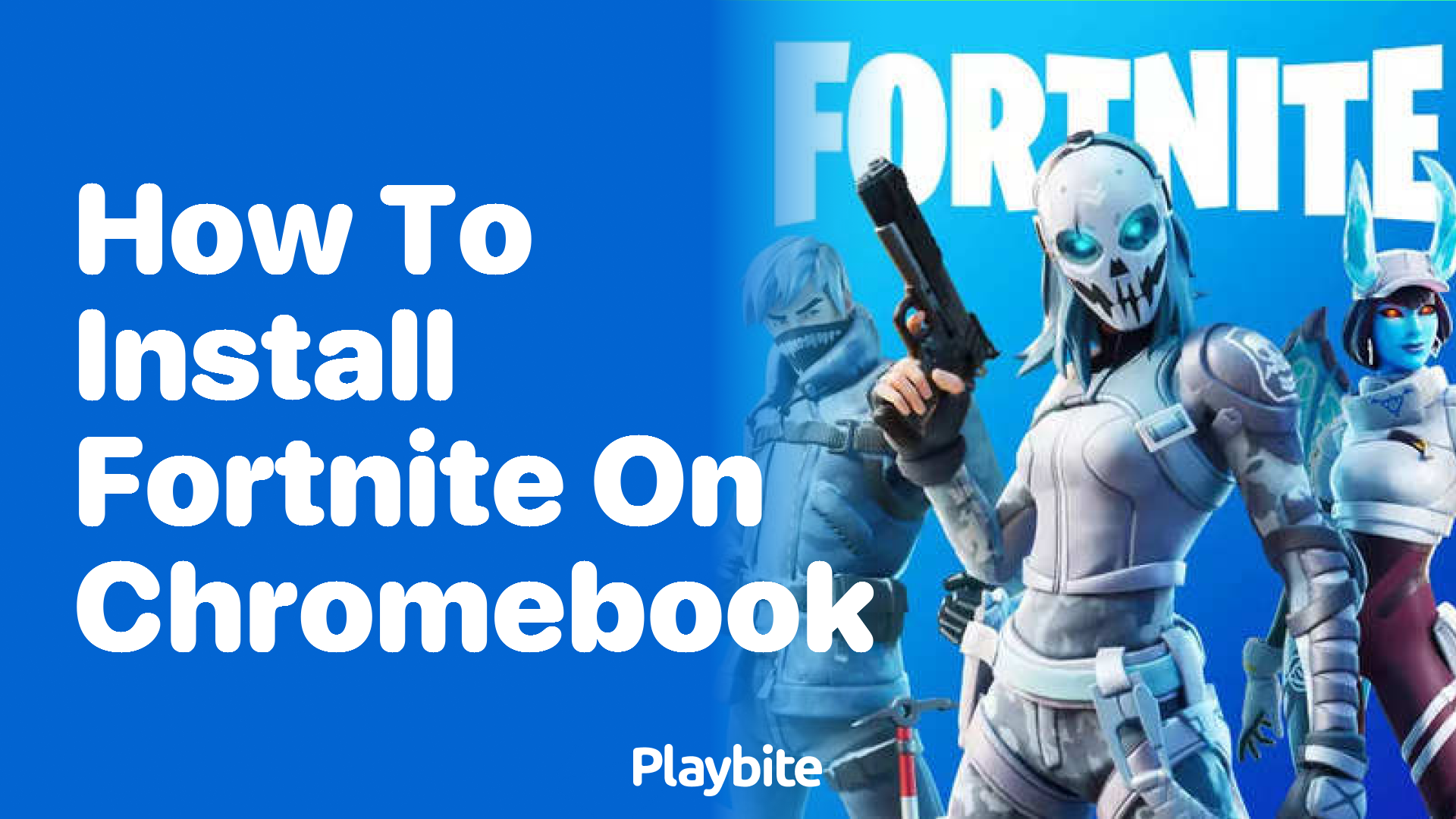The image is a computer-generated advertisement for Fortnite, primarily featuring a bright blue gradient background with a faded white overlay on the right side. Dominating the upper left part of the image are bold white letters that read "How to Install Fortnite on Chromebook," with "Playbyte" displayed prominently below it. Across the top of the image is a large "Fortnite" banner. Positioned to the right side of the image are three distinct characters from Fortnite. 

The central figure appears to be a woman adorned in silver armor and holding a large black gun. She has a blue-colored face and is wearing a white mask. To her left stands a character with a masked face, light-colored hair, and a vest, with a pickaxe attached to their right leg. On the right is another female character sporting red pants, a silver cropped sweatshirt, and a hat with bunny ears, emphasizing her blue skin. The overall composition highlights the vibrant and dynamic characters against the simple blue backdrop.